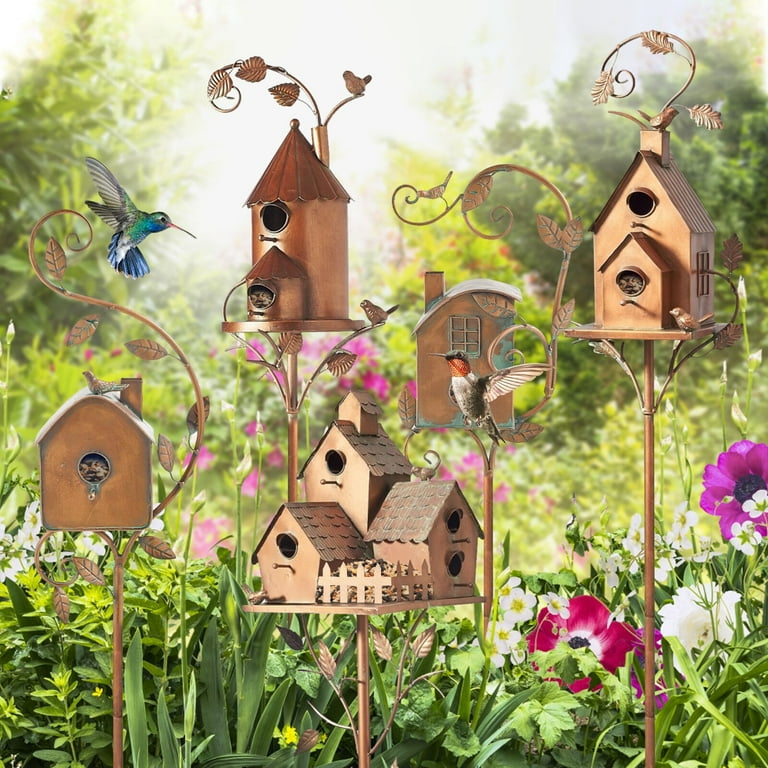This AI-generated image features an intricate and picturesque scene of five detailed birdhouses in a lush garden setting. The foreground, more sharply focused than the softly blurred background, showcases these copper-colored birdhouses, each exquisitely designed, sitting atop vine-like metal rods. From left to right, the first birdhouse is minimalistic with a single entrance hole, a chimney, and a curling vine ornament. Next is a multi-story birdhouse with a triangular roof and circular base, resembling a silo, containing two openings. The central birdhouse is a complex structure combining three birdhouses into one: a double-story house with a small picket fence connecting to a larger two-story house, both with multiple entrances. The fourth birdhouse features a single hole and a faux window, while the final house on the far right mirrors a church steeple design with two entrances. The garden setting behind them is lush with green and yellow hues, dotted with flowers and overgrown foliage, resembling an idyllic oasis. Illuminated in soft, overcast sunlight, the scene also includes a vibrant blue hummingbird on the left and a red and brown robin-like hummingbird on the right, captured in stunning stop-action detail.